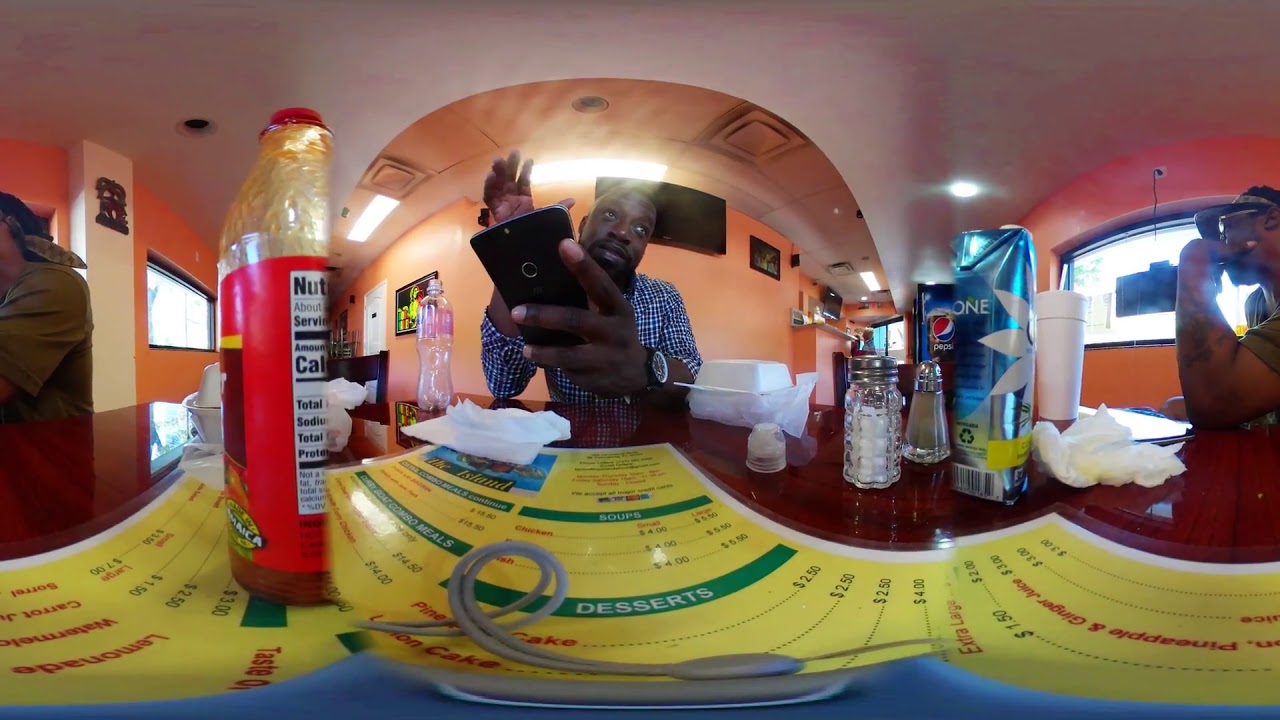The photograph captures a cozy restaurant scene with a distinctive fisheye-like filter, giving the image a curved, spherical appearance. At the center of the image, an African-American man, dressed in a blue and white checkered button-up shirt, sits at a brown wooden table, his hands resting on the surface. He holds a mobile phone in the same hand that displays a watch. The table is scattered with laminated menus, various drinks, including a partially visible hot sauce bottle, a Pepsi bottle, a coconut water pouch, and a Styrofoam cup. There are also salt and pepper shakers and white napkins visible on the table.

To the right, another African-American man is seated, wearing glasses and possibly a visor. He has one arm propped up on the table with his hand touching his mouth, showcasing a tattoo on his hand. 

The background reveals light orange—or peach-colored—walls adorned with paintings and a mounted TV display. Overhead, lights hang from the ceiling, illuminating the scene. Through the windows, white light filters in, accentuating the warm, homey atmosphere of the restaurant.